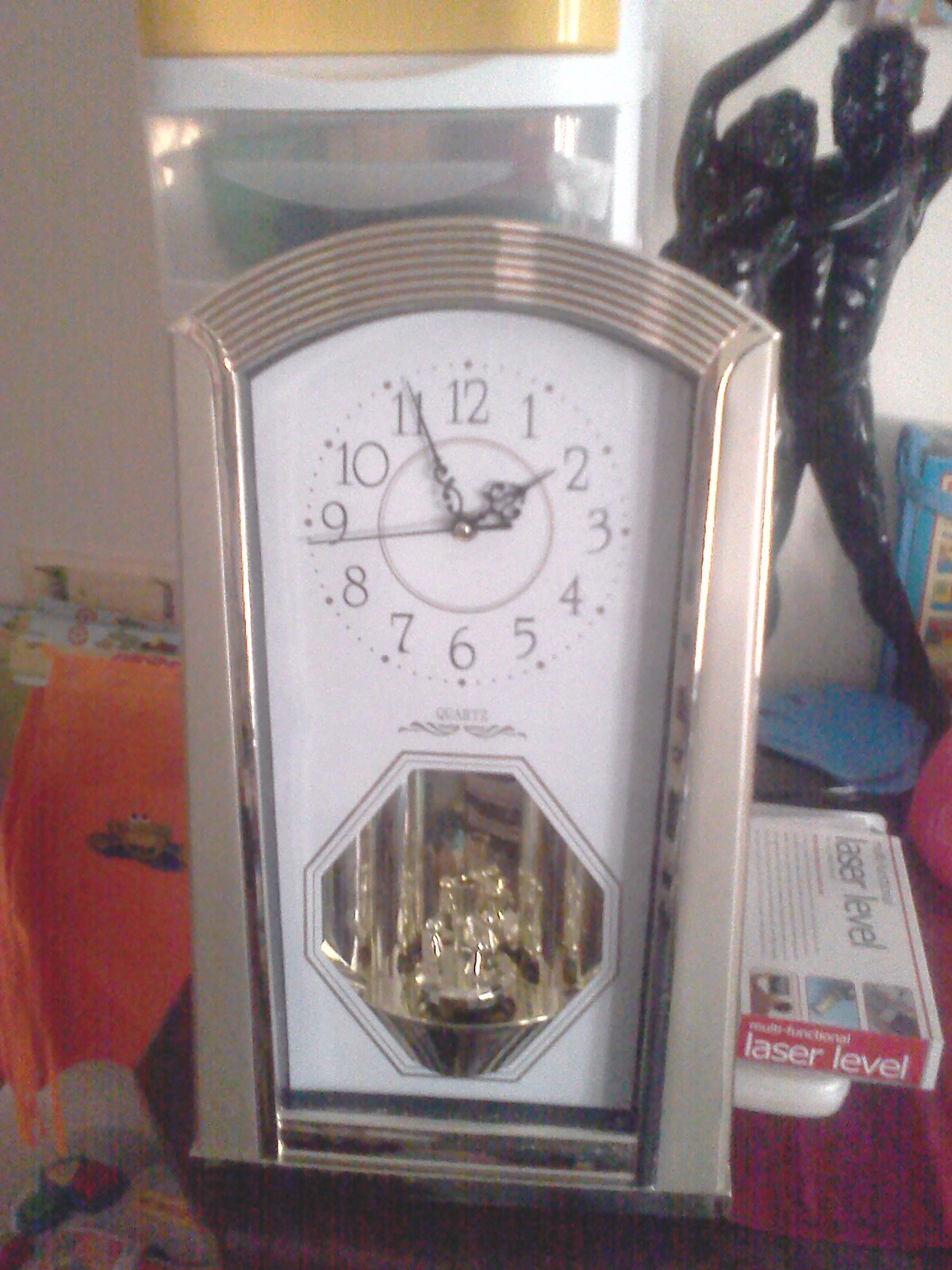The image features a variety of objects with the focal point being an intricately designed clock placed prominently in the center. The clock boasts a distinctive shape, with a rectangular body that transitions into a semi-circular top. The clock face is white, and it is encased in a sleek silver border. The numbers on the clock are black and intriguingly arranged to run counterclockwise. The time is indicated by three black hands. At the bottom of the clock face, the word "QUARTS" is displayed in uppercase letters. Below this, the name is spelled out as "Q-U-A-N-T-Z" in a similar fashion. Further below, an octagonal shape is depicted. In the heart of the clock, a golden object adds a touch of elegance. Background details suggest the presence of additional objects, enhancing the sense of depth and complexity in the overall composition.